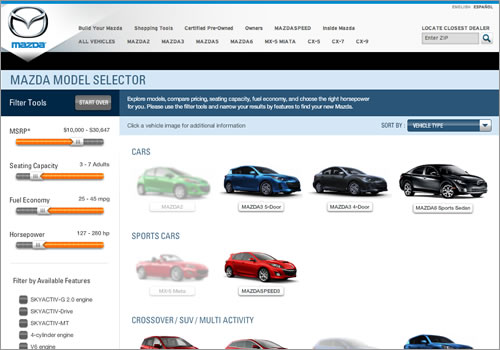Screenshot of a Mazda Car Dealer Website Interface

In this detailed screenshot of a Mazda dealer's website, the top-left corner prominently features the Mazda logo, with the word "Mazda" written in blue beneath it. The top navigation bar includes clickable options for various models such as "All Vehicles," "Mazda 2," "Mazda 3," "Mazda 5," and "Mazda 6," allowing users to easily browse different car types.

Directly below the navigation bar is a blue section labeled "Mazda Model Selector" and "Filter Tools," offering various filtering options. A "Start Over" button is conveniently located within this blue bar, enabling users to reset their selections and filter criteria.

Beneath the blue bar, the interface displays filters for users to refine their search results by parameters like price, seating capacity, fuel economy, or horsepower. This helps potential buyers customize their search according to their needs.

In the bottom right section of the screenshot, there is a white background showcasing multiple Mazda cars. These cars are aligned, facing towards the right, and are organized into rows. The top row features models like the Mazda 3, 5, and a sports sedan, displayed in colors such as green, blue, and black. The middle row highlights various sports cars. Although the bottom row is partially visible, it is indicated as containing crossover SUVs and multi-activity vehicles, with just the tops of these cars peeking into view.

Overall, the interface appears user-friendly and visually appealing, designed to assist prospective buyers in effortlessly navigating through Mazda's diverse vehicle offerings.